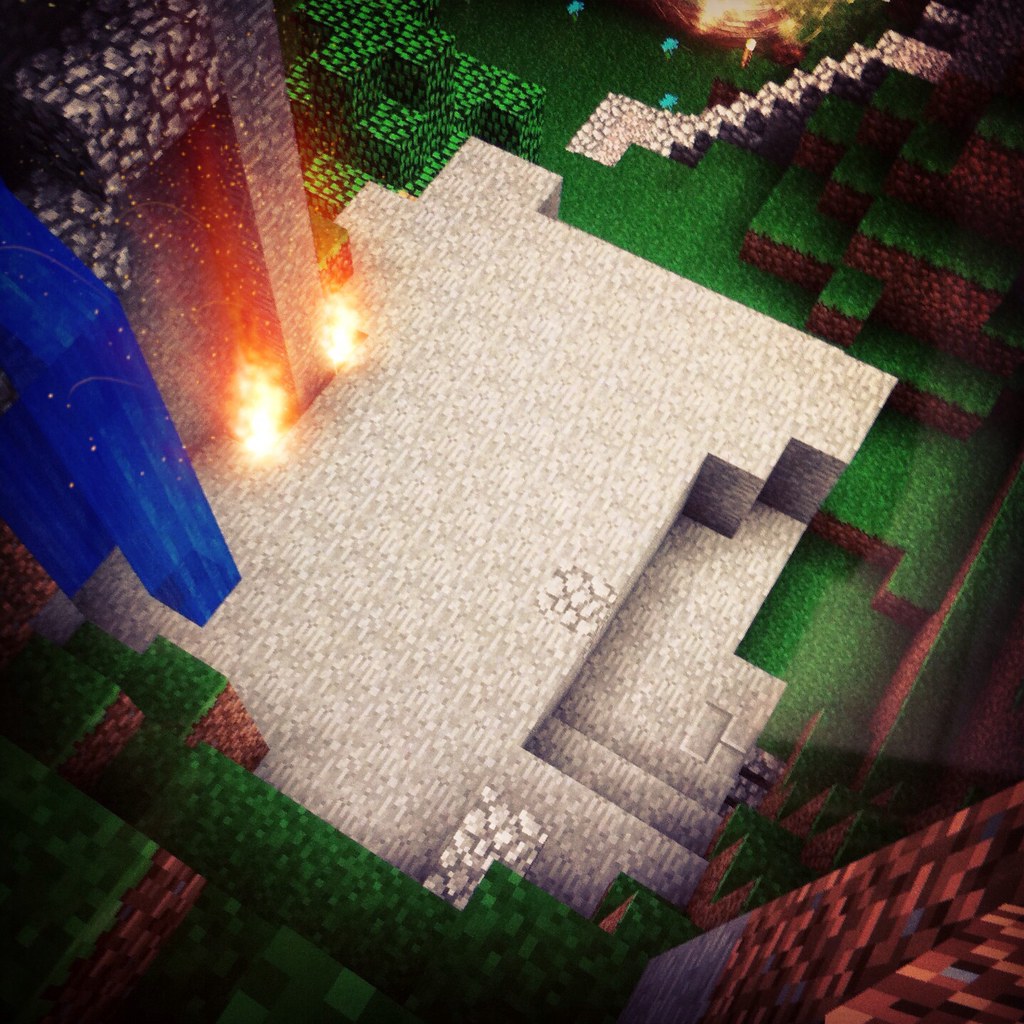A computer-generated image depicts an aerial view of a modern outdoor patio designed with geometric precision. The main stage of the setting is a rectangular platform adorned with a lilac and white pebble-like texture that creates a repeating pattern. To the right, two steps lead down to a slightly lower level. On the left side of the upper level, a tall column made of peach-colored brick with black and white detailing at the top stands prominently. Adjacent to it is a tall royal blue post, accompanied by another post behind it. The entire area is bordered by artificial green bushes and cubic formations. Around the perimeter, sections of exposed earth with patches of green vegetation add a natural touch. The design predominantly favors straight lines and angular shapes, with the exception of two bright white lights featuring red and orange accents, positioned on either side of the peach-colored column, resembling flames.